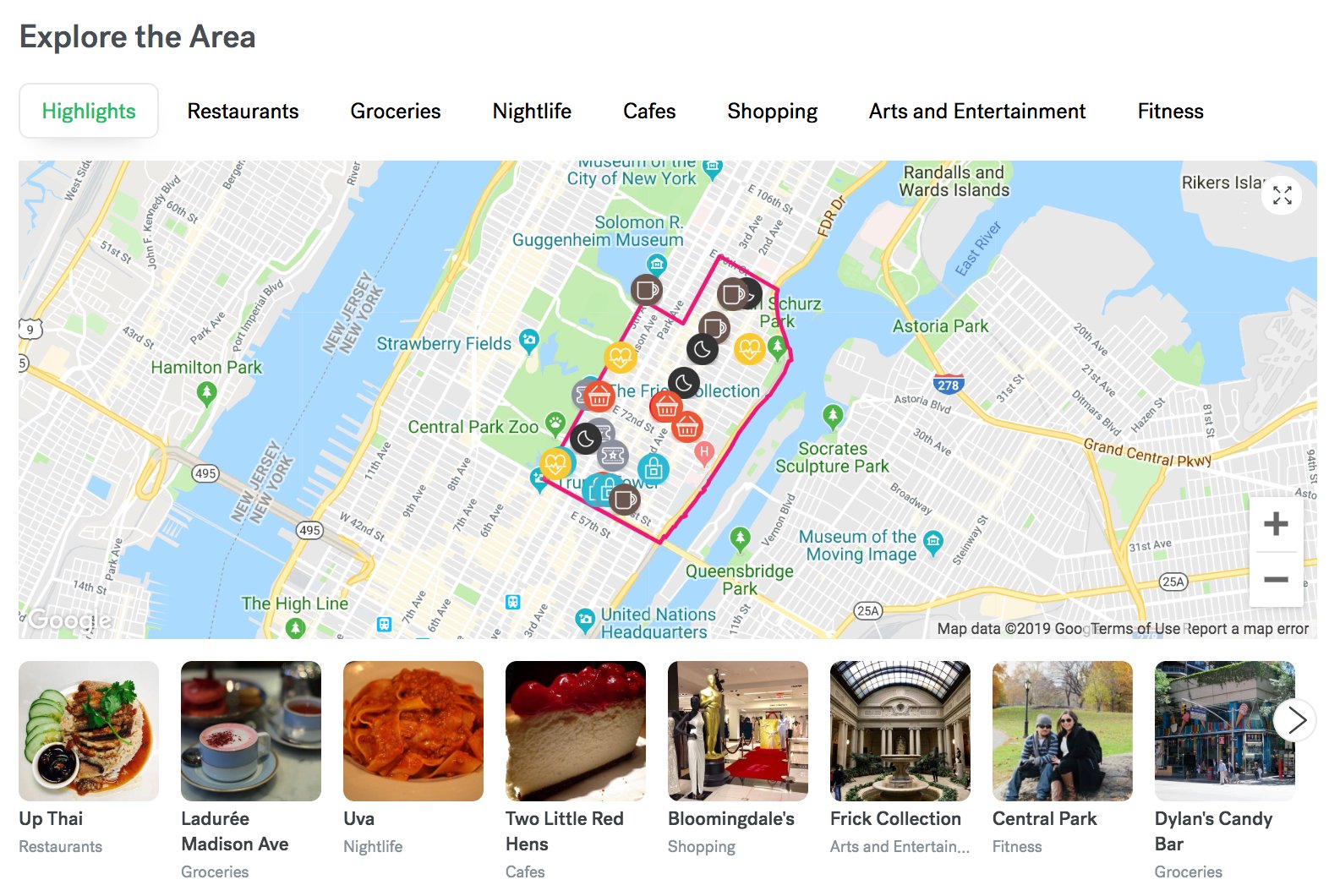This image features a detailed view of the 'Explore the Area' section of a website, focused on a vibrant section of Manhattan, New York City. At the top, there is a white box with categories highlighted in green, including 'restaurants,' 'groceries,' 'nightlife,' 'cafes,' 'shopping,' 'arts and entertainment,' and 'fitness.' Dominating the interface is a large, interactive map that spans horizontally across the screen, marking a densely populated area rich in shopping, dining, and nightlife options.

Beneath the map, there are representative images and specific place names that offer a glimpse into local attractions. These include 'Ladurée' associated with restaurants, 'Madison Avenue' known for groceries, 'Uva' for nightlife, 'Two Little Red Hens' as a cafe option, 'Bloomingdale's' for shopping, 'The Frick Collection' for arts and entertainment, 'Central Park' for fitness activities, and 'Dylan's Candy Bar' listed under groceries.

Additional functionality on the map includes plus and minus signs, allowing users to zoom in or out for a more detailed view or broader perspective, enhancing the ease of navigating and understanding the area. Directions for reaching various destinations are also available, ensuring that whether entering or exiting, users can find their way smoothly.